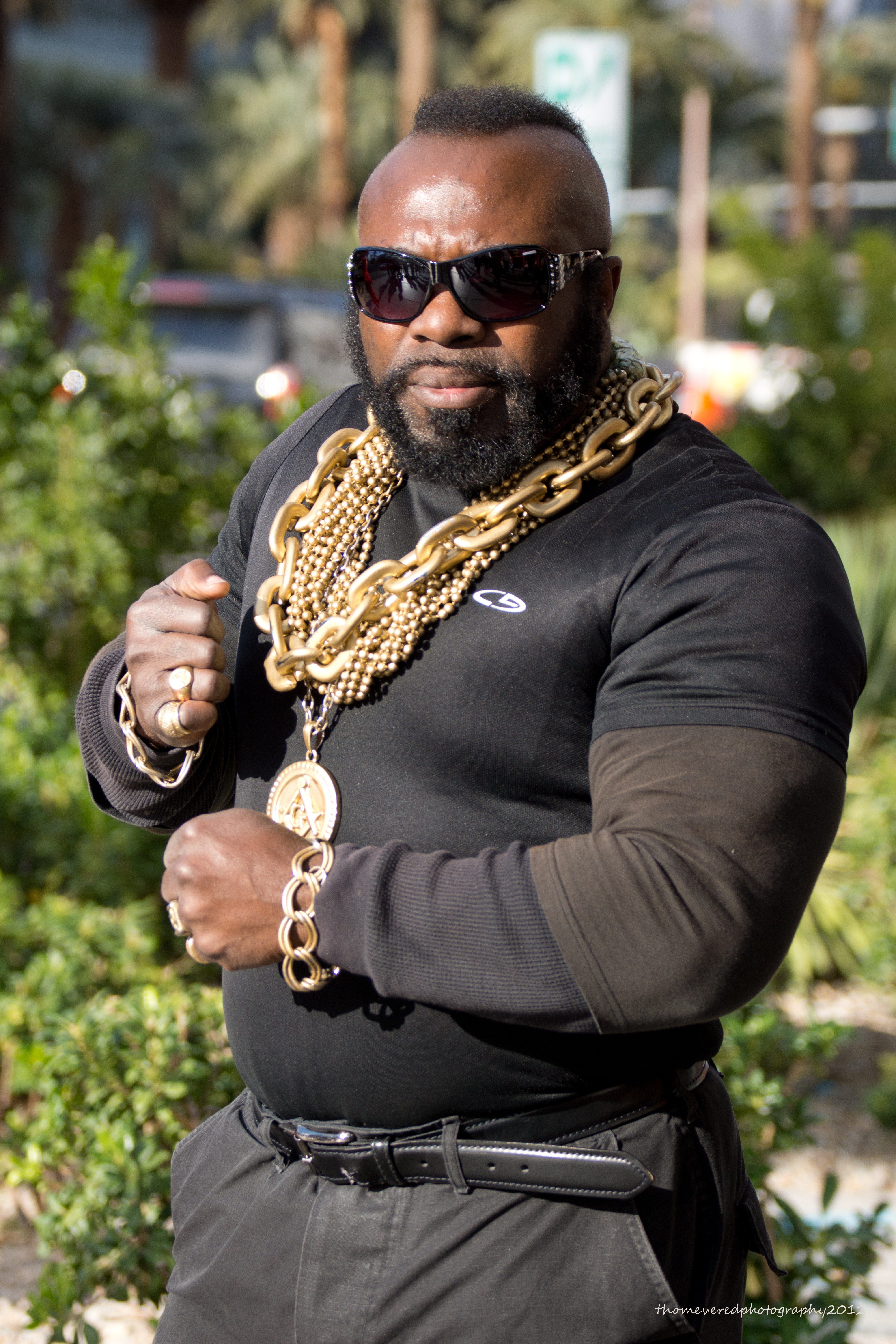The photo captures a muscular black man, likely Mr. T, standing outdoors in what appears to be a garden or courtyard on a bright day. He is positioned centrally in the image, directly facing the camera. He sports a black long-sleeve shirt with a symbol on the right side, and gray pants held up by a dark belt. Adorning his neck are multiple large gold chains, and he wears gold bracelets on both wrists. His distinctive look includes a mohawk, dark sunglasses, a mustache, and a well-trimmed beard. Surrounding him, the background is filled with various bushes and small trees, further indicating the outdoor setting. Also visible are a couple of signs and a vehicle with lights on, but no text is present in the image. The color palette includes shades of black, white, gray, brown, gold, green, and red. His arms are positioned with one across his belly and the other flexed towards his chest, enhancing the impression of his muscular build.